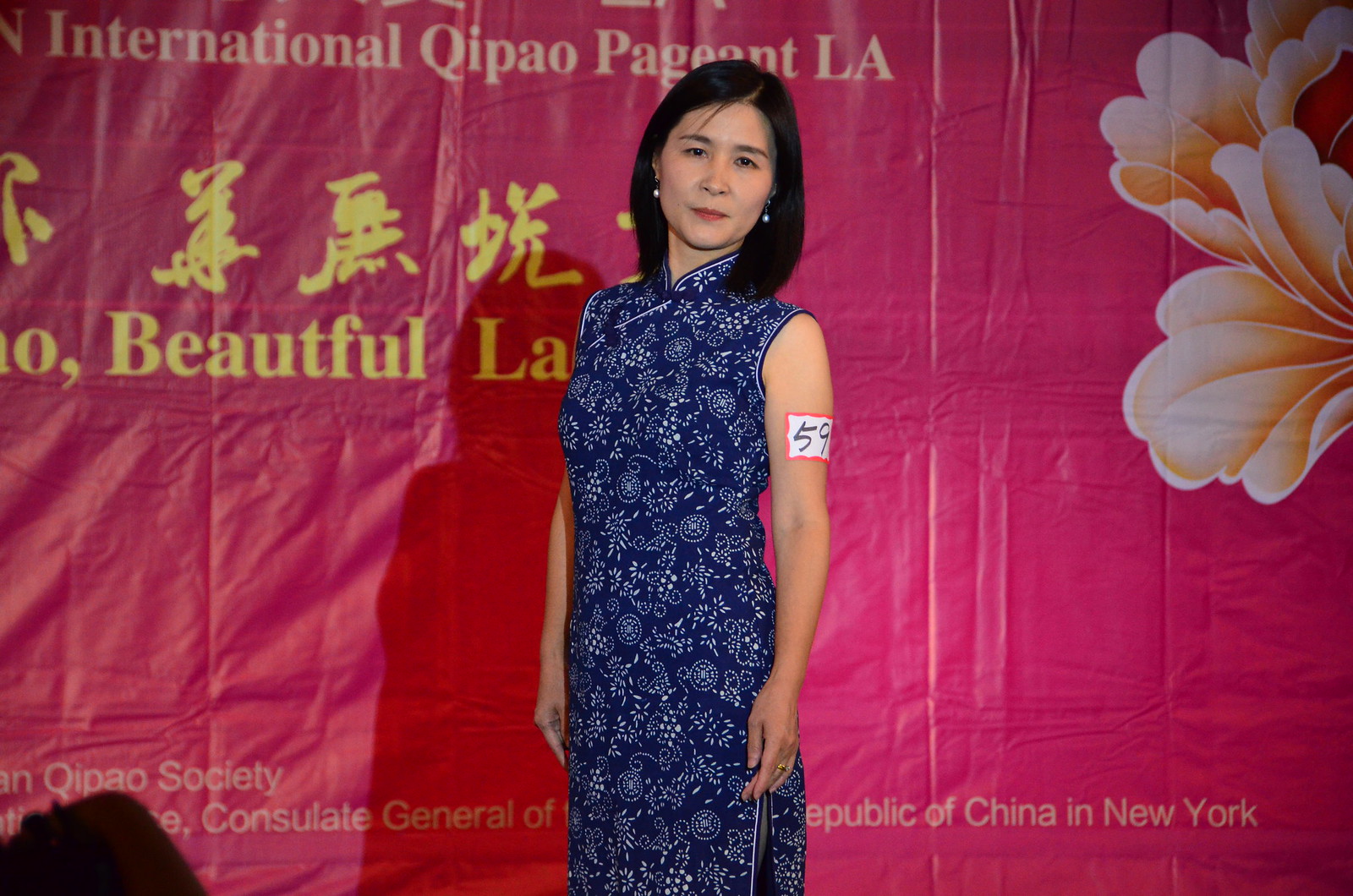In the image, we see an Asian woman posing in front of a red backdrop adorned with several elements. She is wearing a high-neck, short-sleeved, blue dress with white floral and various intricate designs. Her black hair is styled to neck length, and she accessorizes with earrings and a ring on her left hand. On her left arm, there is a sticker with a red border and white background, displaying the number "59." The backdrop features a drawing of a flower at the top right corner and a mix of English and Chinese text. From left to right, the English text reads: "International Qipao Pageant LA" followed by some Chinese characters, the word "beautiful," and at the bottom, "Qipao Society Consulate General of Republic of China in New York." The composition and attire suggest that the image is likely taken during a fashion show or cultural event.